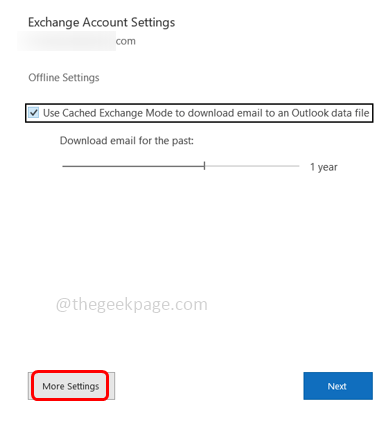This image, captured on a cell phone, displays the settings screen for an Exchange account in Microsoft Outlook. At the top, the header "Exchange Account Settings" is visible. Directly below, there's a section obscured by a blurred rectangle to protect sensitive information, though part of a domain ending in ".com" is still partially visible.

The screen then lists "Offline Settings," under which there's a checkbox with a blue check mark labeled "Use Cached Exchange Mode to download email to an Outlook data file." Following this, the screen states "Download email for the past:" accompanied by a slider that stretches across the display, ending at "1 year," indicating the preset duration for email downloading.

Further down, a placeholder text "at thegeekpage.com" is visible, potentially from a tutorial or help page source. Near the bottom, a "More Settings" button appears, highlighted with an additional red rectangle drawing attention to it. Finally, a blue "Next" button is situated in the lower right corner of the screen, ready for the user to proceed with the configuration process.